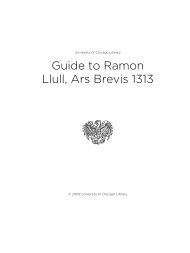The image features a simple, black-and-white cover for a publication, dominated by a stark, white background. At the top, in prominent black letters, the title reads, "Guide to Ramon Llull, Ars Brevis 1313," with the phrase split across two lines: "Guide to Ramon" on the first line, and "Llull, Ars Brevis 1313" on the second line. Notably, only the first letter of each word is capitalized, except for the "t" in "to."

Centered below the title, there is a logo depicting an eagle with wings spread wide, facing towards the left. This crest is the central visual element on the cover. Above the title and below the eagle image, there is some text that is so minuscule it is unreadable. The entire design, from the textual elements to the eagle logo, is rendered in black ink against the untouched white of the paper, maintaining a clean and minimalist aesthetic.